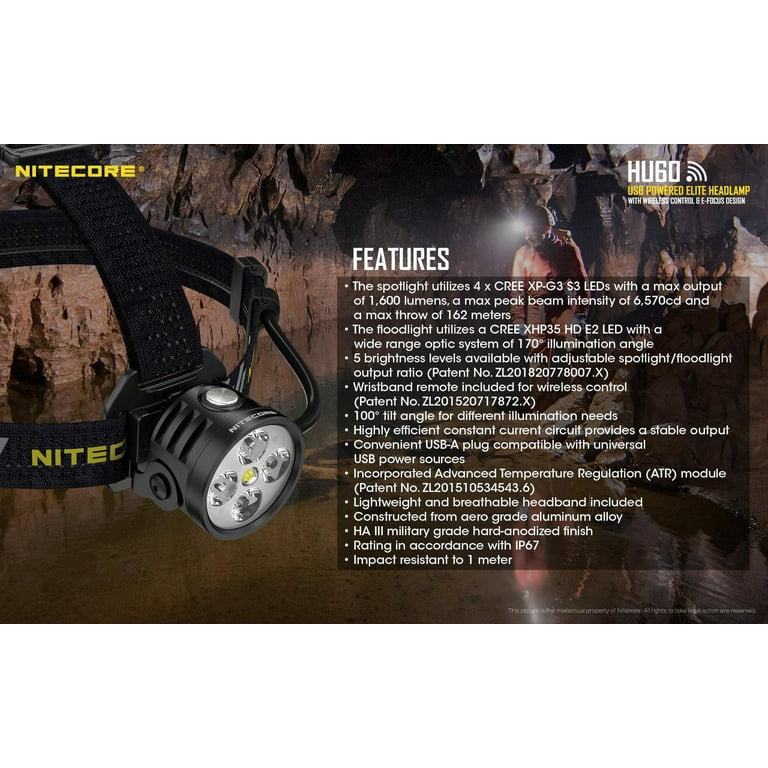The advertisement showcases the "Nitecore HU60 USB Powered Elite Headlamp," with its striking features and high-performance specifications. Prominently on the left side, the headlamp is depicted with black straps that wrap around the head, branded with "Nitecore" in yellow both at the top and along the strap. The headlamp's front displays four circular lenses, powered by Cree XPG3 S3 LEDs, delivering a maximum output of 1,600 lumens, a peak beam intensity of 6,570 CD, and a beam throw reaching up to 162 meters. Additionally, it boasts impressive features such as wireless control and an e-focus design. The background subtly merges into an image of a cave, showing a man wearing the headlamp and highlighting its brightness. The top right corner of the ad reads "HU60" in white and yellow, along with key phrases like "USB Powered Elite Headlamp," "with Wireless Control," and "e-focus design." The right side features a semi-transparent dark field detailing the headlamp's robust qualities, such as impact resistance up to one meter and IP67 rating for water and dust resistance. The comprehensive list of features emphasizes the headlamp's advanced and durable design, confirming its utility for demanding environments.